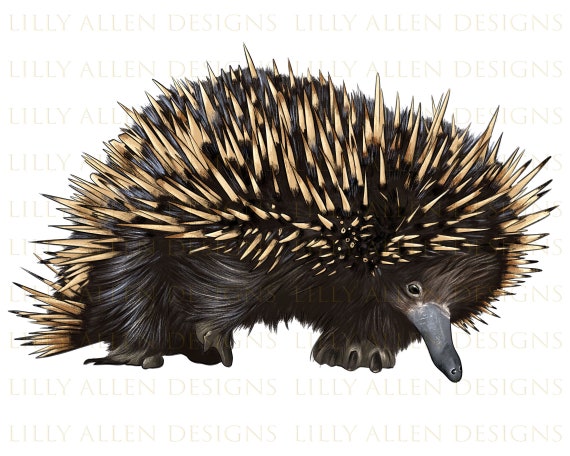This detailed artwork portrays a porcupine with distinct characteristics, set against a stark white background. The porcupine features a mass of ominous, off-white quills that stand out sharply from its black fur. Its long, slender snout is gray, accentuating a curious and pointed appearance, with visible nostrils at the end. The creature’s small dark eye peers out, and its black claws look notably sharp and long. The design highlights sections of the porcupine’s anatomy, such as the dark fur on its underbelly and paws which appear softer in contrast to the quills. The image is subtly marked with the repetitive text "Lily Allen Design" in light font across the background, indicating the artwork's creator.